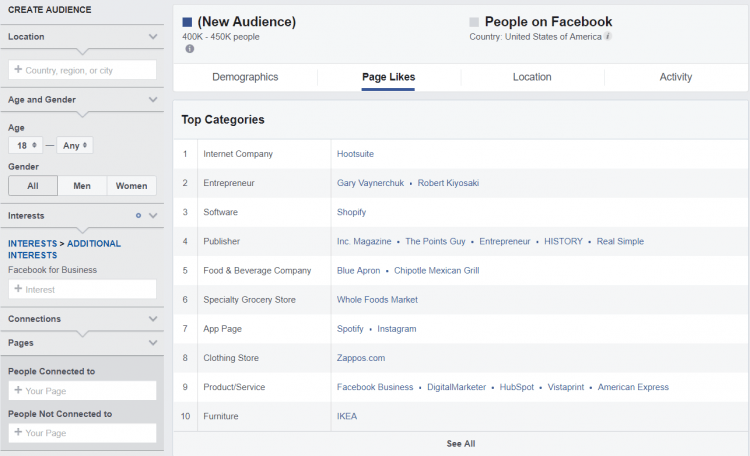The image depicts a detailed view of a Facebook analytics page designed for marketers and page administrators. At the top of the page, users can see a section highlighting "New Audience," while the "People on Facebook" option is not highlighted. Below this, there are four tabs labeled: "Demographics," "Page Likes," "Location," and "Activity." Currently, the "Page Likes" tab is selected, revealing additional data related to it.

Under the "Page Likes" section, a list of the top ten categories is displayed. The first column lists category names such as "Internet Company," "Furniture," and "App Page." Adjacent to this, the second column showcases the leading websites or apps within each category. For example, "Shopify" is listed as the top site in the "Software" category, and "IKEA" ranks highest in the "Furniture" category.

On the left side of the page, there is a "Create an Audience" section, featuring a series of customizable windows. This allows users to create tailored audiences by selecting various demographic factors including age, gender, interests, and connections. This setup facilitates targeted audience creation for marketing and engagement purposes.